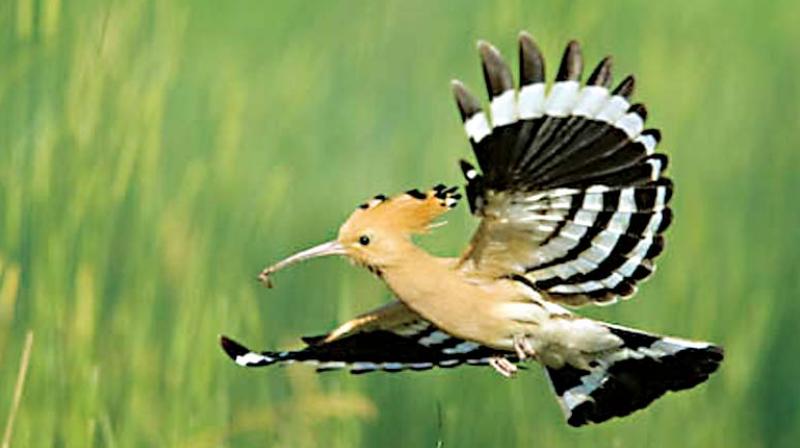This photograph captures the dynamic scene of a large bird in mid-flight against a backdrop of tall, out-of-focus green grasses with yellow tips. Dominating the left, center, and right side of the image, the bird's wings are elegantly outstretched, revealing a striking pattern. The upper body and head of the bird are primarily a yellowish-brown, complemented by a distinctive crest on its head with black flails. It has a white underbody that extends towards its tail, which showcases alternating black and white stripes with the tips of the tail feathers being black. The bird’s wings feature intricate black and white striping, with the tips of the feathers dipped in black, resembling the fan of a delicate hand fan. Its long, pointed white beak clutches a brown, worm-like insect at the tip, while its black eyes survey its surroundings. The detailed pattern on its wings and tail, along with the bird's poised capture in flight, make for a visually stunning and intricate portrait set against a blurred, grassy background.